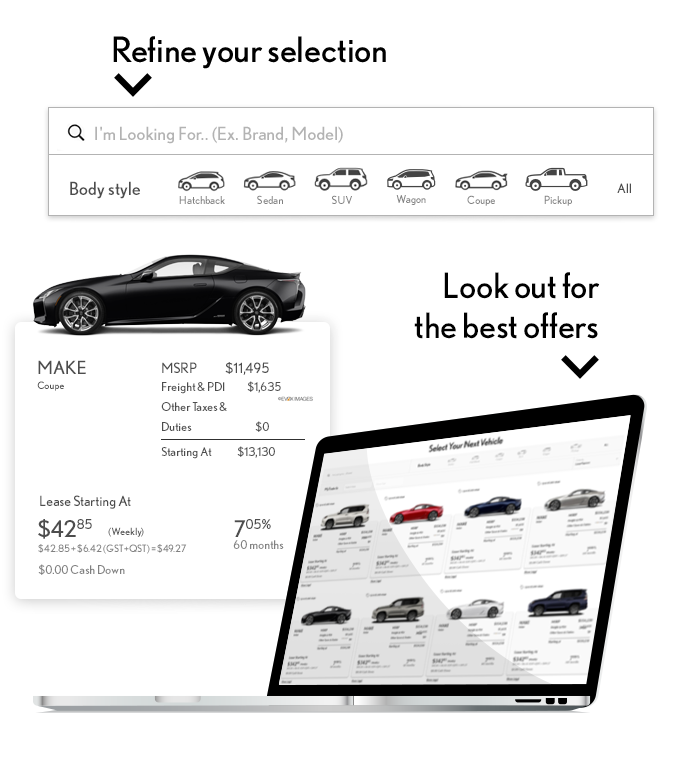**Image Caption: Refine Your Selection Mockup**

At the top of the web page mockup, there is bold black text that reads "Refine Your Selection" accompanied by a black down arrow. Below this, a search bar is positioned inside a rectangular box on the left-hand side. The search bar features a black magnifying glass icon, and the placeholder text in gray reads, "I'm looking for (e.g., brand, model)."

Underneath the search bar, there is a section labeled “Body Style” in black text. This section displays various vehicle types with corresponding images: a small SUV labeled "Hatchback," a maples sedan labeled "Sedan," followed by other body styles including SUV, wagon, coupe, and pickup. The section ends with an option labeled "All."

In the lower left-hand corner of the page, a black sedan is showcased sitting atop a 3D white box. This box includes details about the vehicle: on the left side, it states “Make: Coupe” and on the right, it lists “MSRP: $11,495,” “Freight and PDI: $1,635,” “Other Taxes and Duties: $0,” and “Starting at: $13,130.” Additionally, on the lower left-hand side of the box, leasing information is provided: “Lease at $42.85 weekly,” and below that in gray text “$42.85 + $6.42 (GST + QST) = $49.29.” The bottom of this section notes “$0 cash down.”

On the right-hand side, the loan rate is specified as 7.05% for 60 months, with an arrow pointing down to a tablet displaying the text “Look out for the best offers.”

The image also includes a laptop with a gray keyboard and a black bezel. The screen displays multiple cars in a row: a silver SUV, a red sedan, a blue sedan, a silver sedan, a black sedan, a dark gray SUV, a white sedan, and a dark blue hatchback.